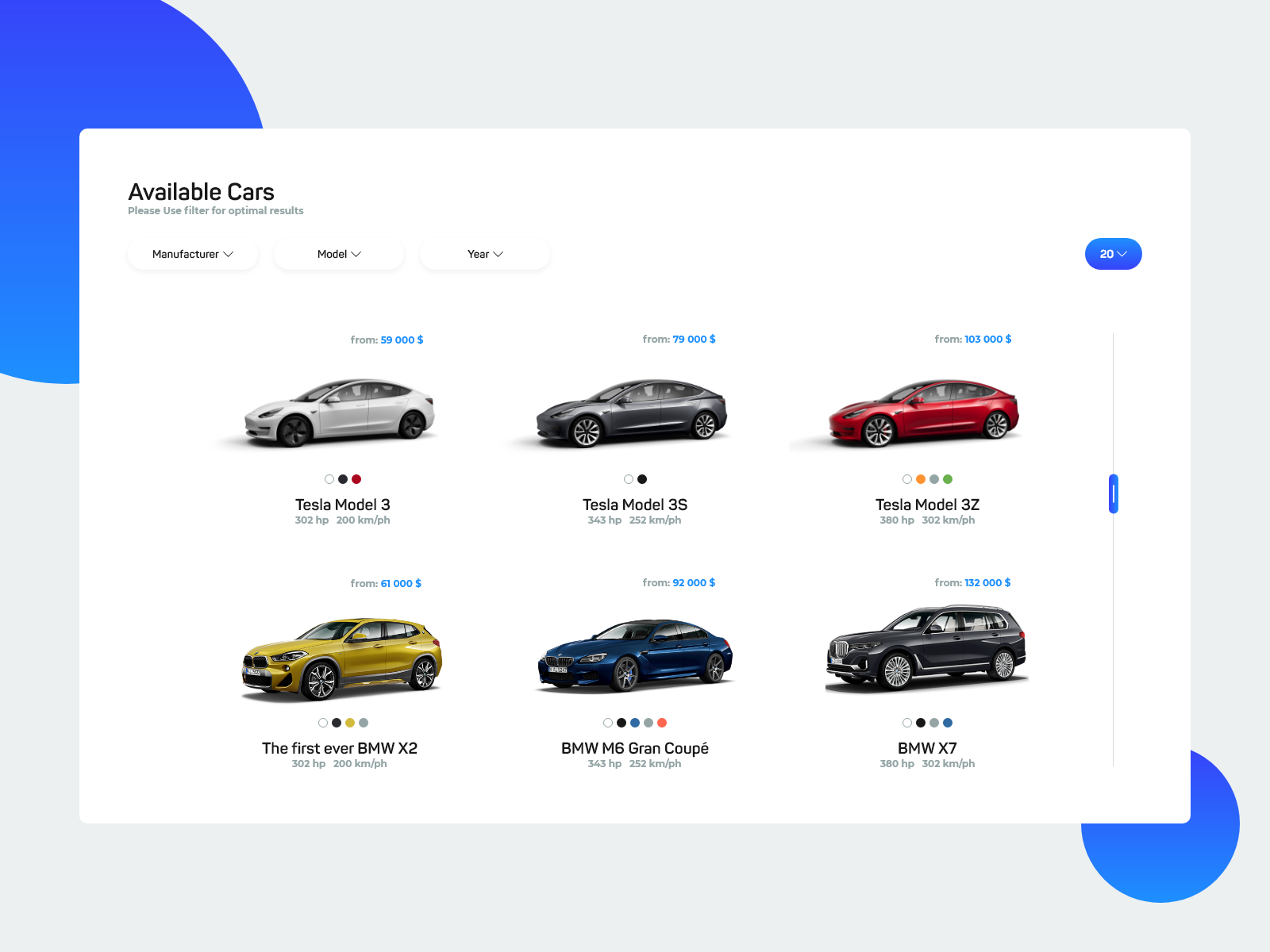This image is a screenshot of a presentation slide. The content of the slide includes a screen capture from a car sales website, displaying various car models available for purchase. The webpage initially appears to be from the Tesla website, showcasing different Tesla car models such as the Tesla Model 3, Model 3S, and Model 3Z. However, upon closer inspection, it becomes evident that the site also lists BMW models, including the BMW X2, the M6 Grand Coupe, and the X7, indicating that this is a multi-brand car sales site rather than just Tesla's. The user, as shown by the scroll bar, is less than halfway down the page of a total of 20 cars available for viewing. Additionally, there are two blue circular elements faintly visible in the background, partially obscured by the main webpage content.